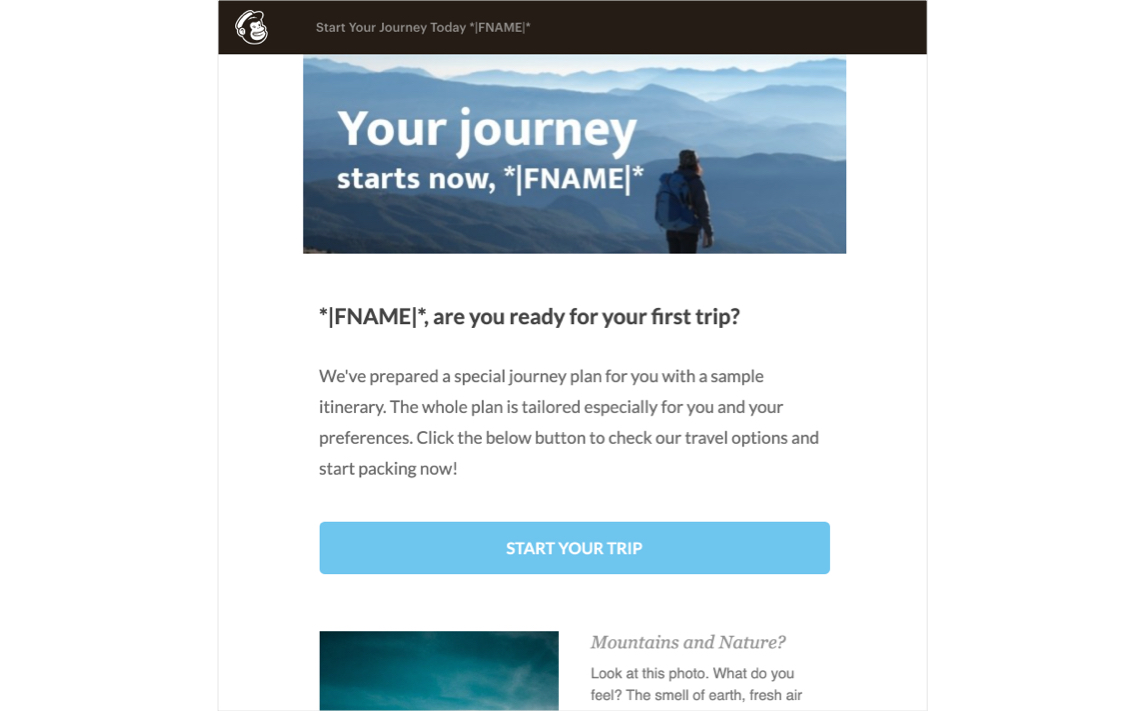The image depicts a MailChimp landing page, identifiable by the iconic chimp mascot wearing a mailman’s hat, located in the top left corner against a black banner that stretches across to the top right corner of the page. Adjacent to the MailChimp icon is the phrase "Start your journey today" in gray font, separated by a line from placeholders labeled "F name" marked by asterisks.

The main body of the page features a white background with a central box containing an inspirational image of a person gazing at a mountainous landscape. Superimposed on this image are the words "Your journey starts now" with the placeholder "F name" included. 

Further down, in bold black font, an asterisk with "F name" is followed by the question, "Are you ready for your first trip?" This is followed by an enticing message: "We've prepared a special journey plan for you with a sample itinerary. The whole plan is tailored especially for you and your preferences. Click the below button to check our travel options and start packing now."

Prominently displayed beneath this text is a blue button with the call-to-action "Start your trip" written in white font. Additional content is partially visible towards the bottom, showing the edge of a blue gradient image accompanied by text on the right that reads, "Mountains and nature. Look at this photo. What do you feel? The smell of earth, fresh air..." The text is cut off, leaving the sentiment incomplete.